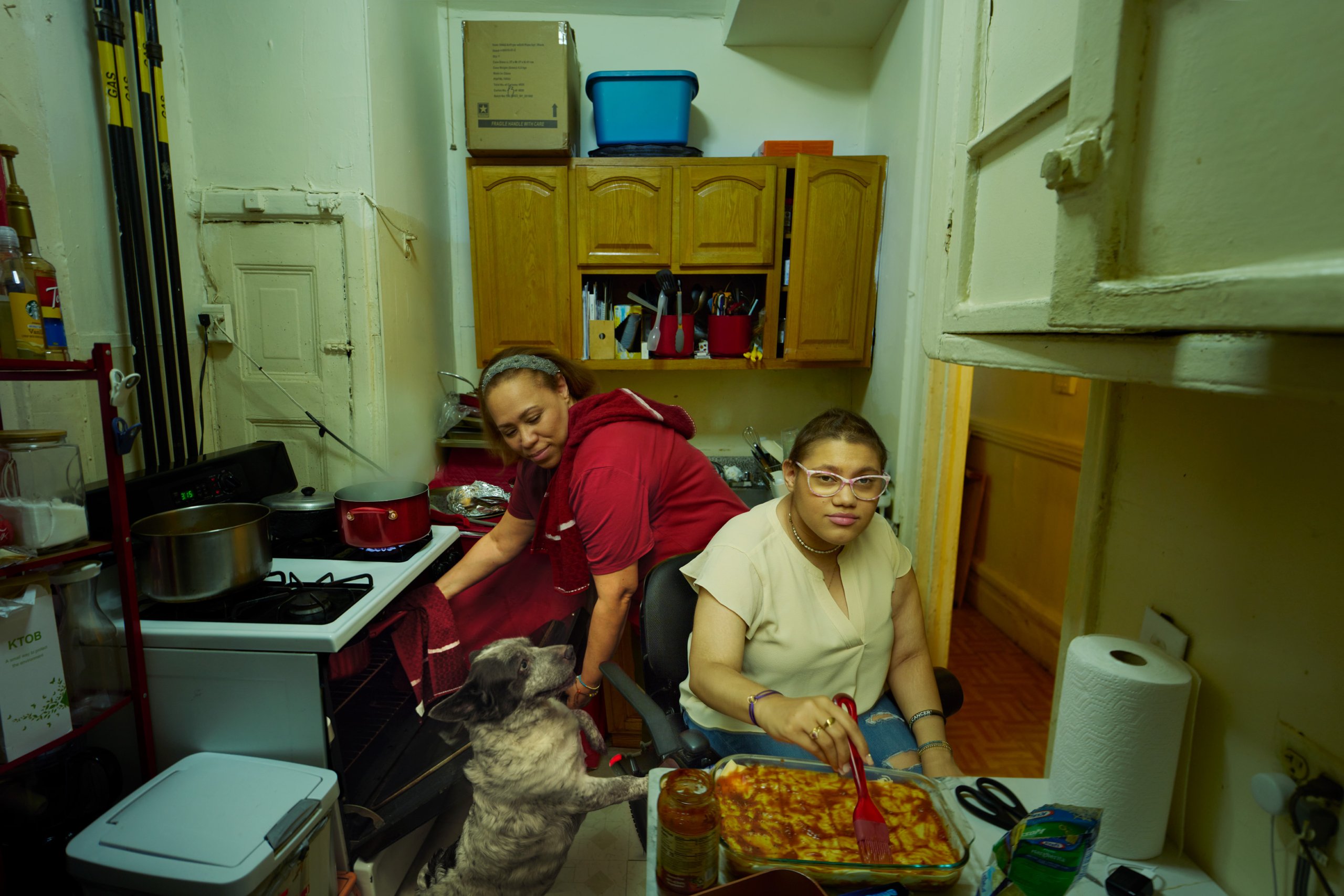In a cramped, bustling kitchen, two Black women are immersed in cooking. The woman in the foreground, with short brown hair pulled back and pink-rimmed glasses, stands at the counter preparing what appears to be a lasagna in a large tin tray. She wears a beige top and holds a red spatula in her left hand, poised to stir or portion out the dish. Standing on its hind legs beside her, a gray and white dog watches intently, seemingly asking for food. Around her, the kitchen is cluttered with various items, including a large roll of paper towels and scissors to her right, and old brown cabinets with a blue bin and a box on top in the background. 

Behind her, another woman in a red blouse with a greenish headband and her hair pulled back bends down to open the oven, which has silver sides and a white top. Pots are boiling on the stove above her, with steam wafting up. The walls of the kitchen are covered in old, peeling white paint, adding to the sense of timelessness and hominess in the space. To the right, there's an entrance or exit way leading out of the kitchen, further emphasizing how packed the space is with all the cooking and activity.